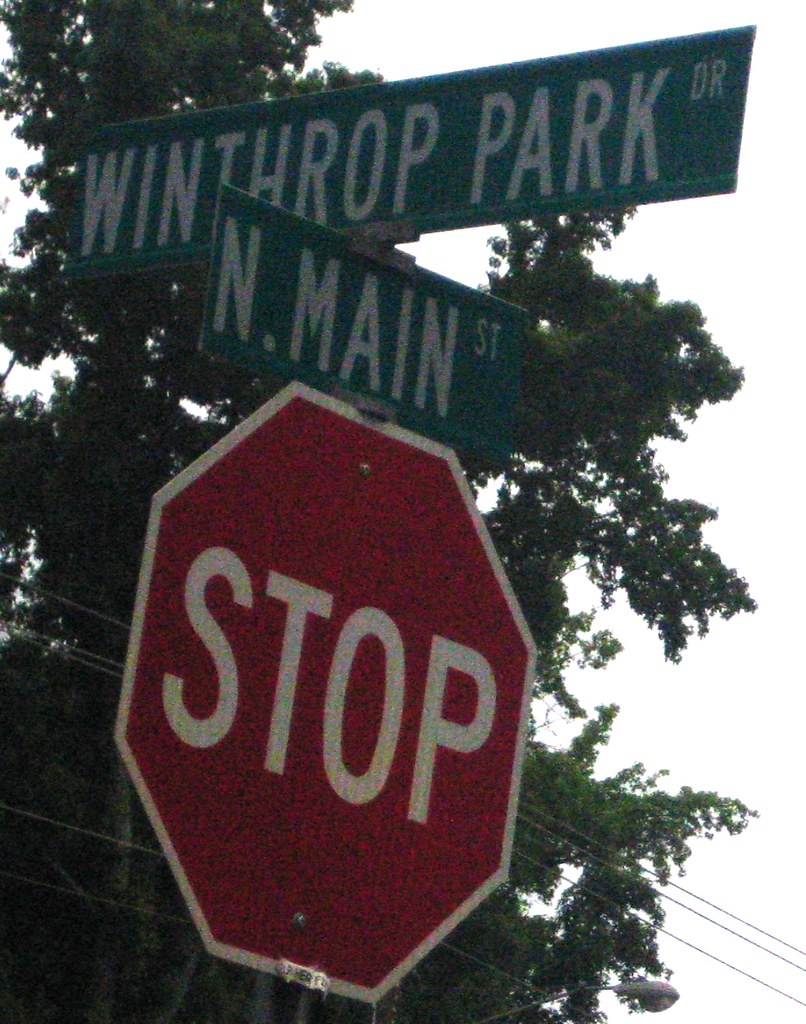In this daytime photograph, the focal point is a prominent red stop sign situated at an intersection. Atop the stop sign are two green street signs; "Winthrop Park Drive" is displayed on the top, while "North Main Street" extends perpendicular below it. A massive tree provides a lush, leafy backdrop, its branches stretching expansively upwards and outward to the right edge of the frame. Power lines also cut across the scene, traversing from the lower left corner towards the bottom right, subtly weaving through the branches in the background.